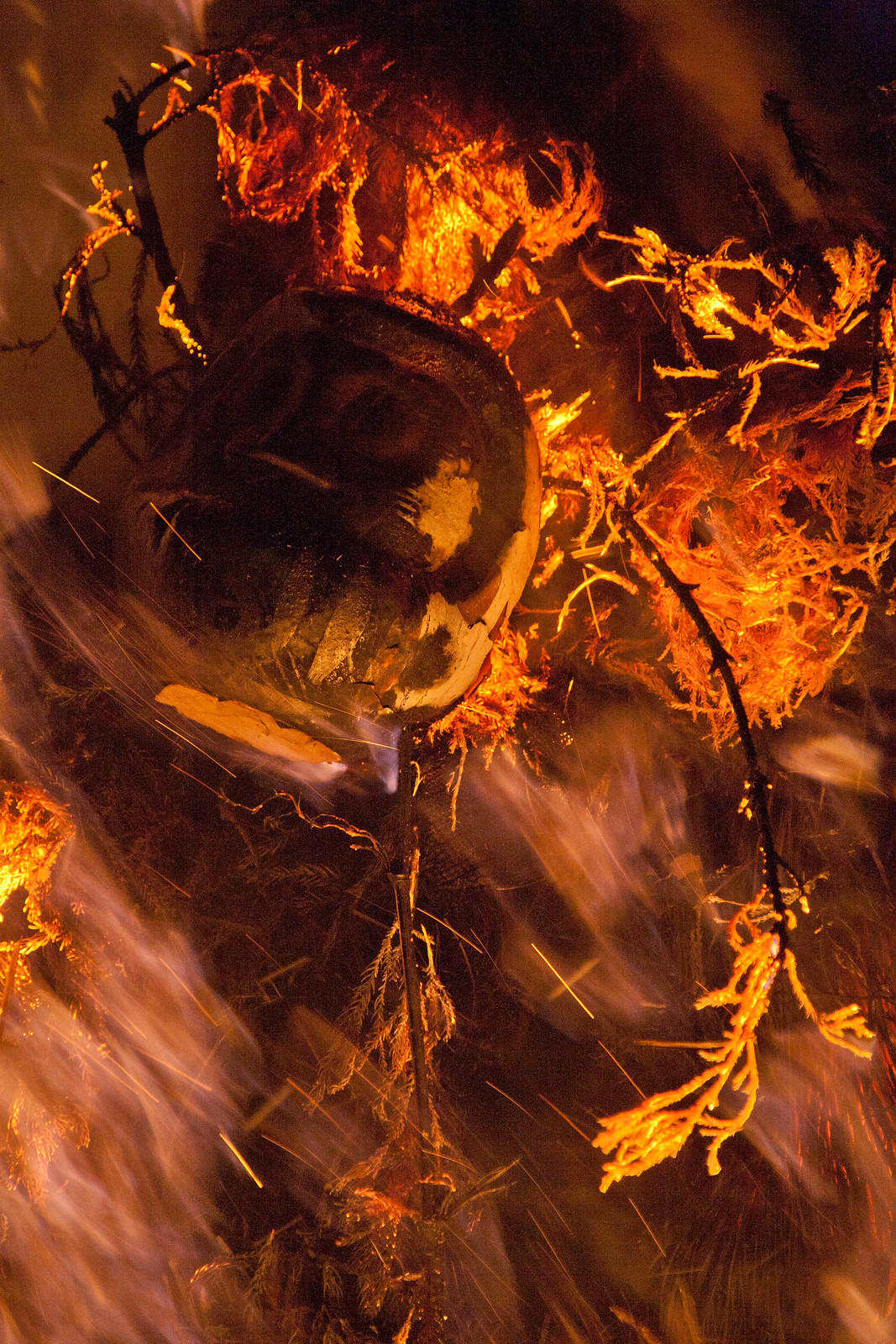This vertically aligned rectangular image, dominated by intense oranges, reds, and browns, depicts a vivid and almost surreal scene of burning plant life. The background is a striking mix of fiery hues and dark shadows, punctuated by streaks and sparks of smoke and light, suggesting a long exposure photograph. The foreground features a tangle of dark brown branches and twigs, some of which, especially near the top, are visibly ablaze, with flames licking upward. Interspersed among the flames are glowing embers that add to the sense of heat and intensity.

Centrally located on the left side is a round, enigmatic object, possibly metallic or organic in nature, that draws the viewer's eye. It has a peculiar appearance with large, contrasting white-around-black eyes and a line for a mouth, giving it a somewhat creature-like vibe, reminiscent of a penguin on a rock. Despite its ambiguous identity, it captivates attention amidst the chaos. The right side and top of the image exhibit the densest concentration of fire, with branches and tendrils hanging down, consumed by flames. The scene is surrounded by patches of bright orange, evidencing the ongoing burn, while the smoky whites and grays add depth and atmosphere to this highly dynamic digital artwork or enhanced photograph.